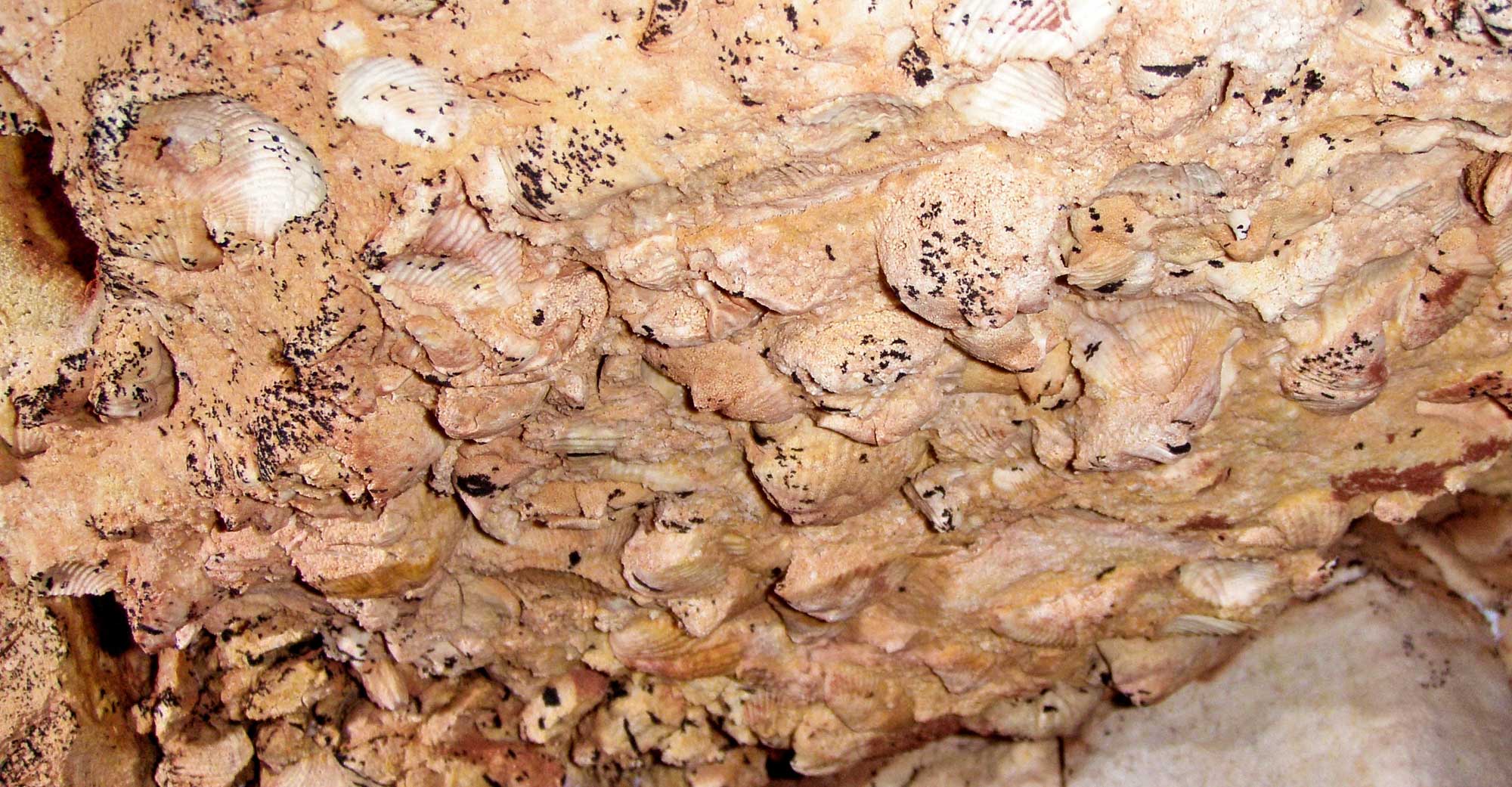This close-up image, taken with bright flash photography, captures the intricate texture of a cave's ceiling, about one foot away from the camera lens. The photograph prominently features a mass of fossilized seashells and crustaceans embedded in the rock, which is predominantly composed of beige to salmon-colored material with striking white shells. The roof of the cave boasts sharp, protruding formations, contrasted by a smooth, gray rock wall visible in the bottom right corner. Interspersed throughout the scene are tiny black specks, which may be small insects or dirt. The photograph lacks any text, allowing the intricate details and organic structure of the cave ceiling to be the primary focus.